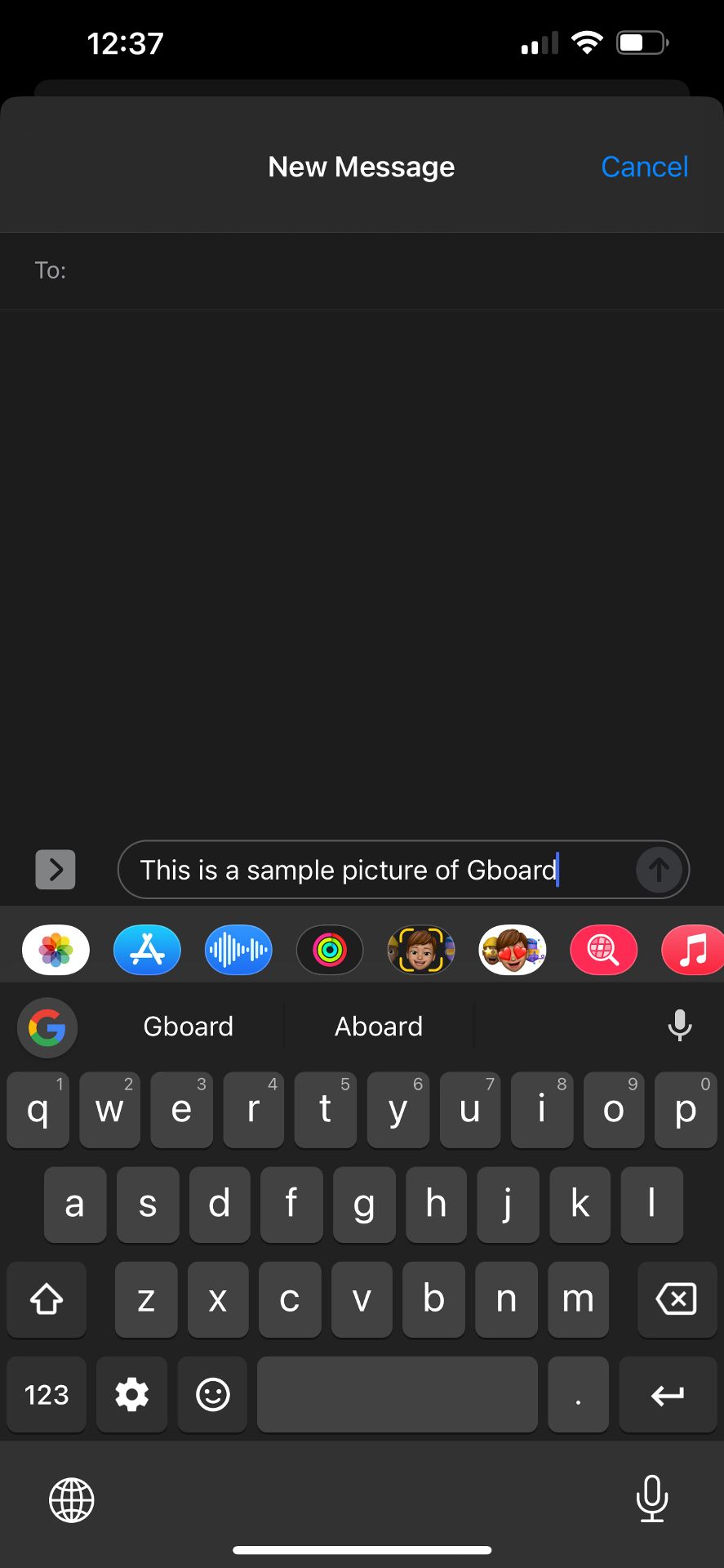The screenshot displays the "New Message" screen on an iPhone at 12:37 PM. At the top, the interface shows the "New Message" header with a "Cancel" option on the right side. The text input area is blank, containing only placeholder text. Below this area, a sample image demonstrates the Gboard keyboard in use. This Gboard keyboard is identified by the distinctive "G" logo located on the left. The keyboard features a standard QWERTY layout along with a predictive text bar. To the right of the space bar, there is a microphone icon for voice input. The interface also includes several app icons such as Photos, App Store, and others, along with a range of emojis and an element resembling Apple Music. The screenshot appears to serve as a demonstration of Gboard's appearance and functionality on an iPhone. It is unclear whether this image is intended for app store promotional purposes or if it was shared on some sort of message board or forum to highlight Gboard's features.